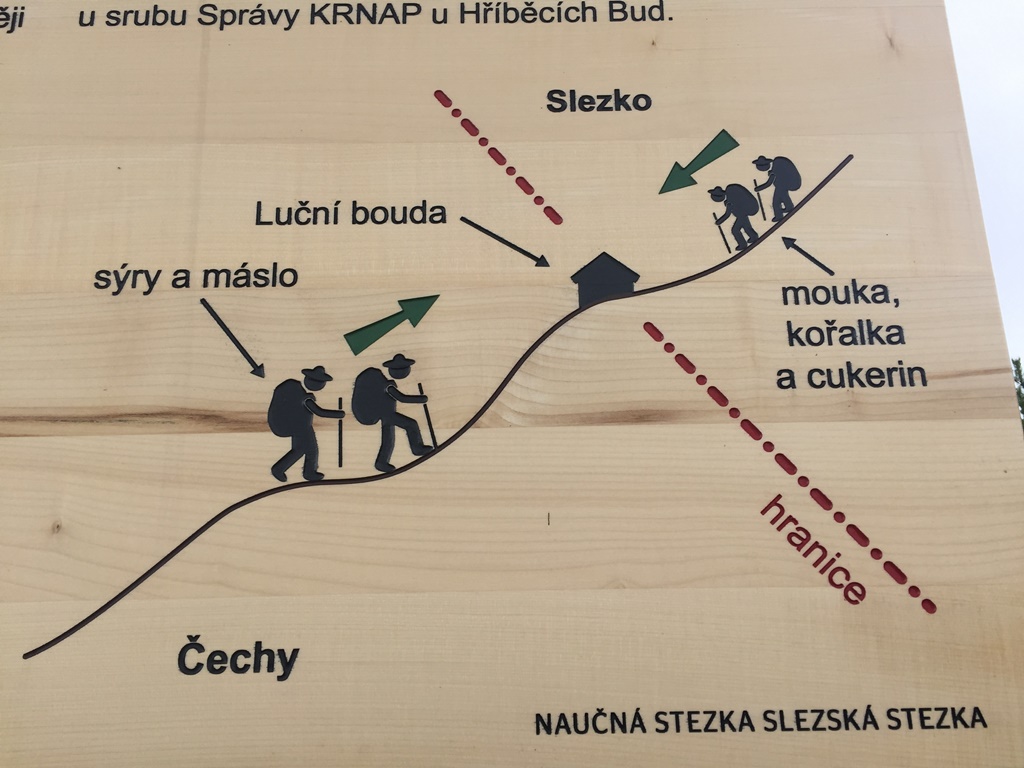This image features an intricately etched diagram on a light-colored wooden board, adorned with non-English inscriptions. The central focus is a curvy, steep black line that zigzags from the bottom left toward the upper right. Along this wavy path, there are simplistic, stick-figure-like illustrations of hikers clad in hats, backpacks, and walking sticks. Two hikers are depicted ascending the hill on the left side of the line, moving towards a small engraved house positioned centrally on the board. Meanwhile, two other hikers are shown descending the hill towards the same house. Green arrows emphasize their direction towards the house, with one arrow pointing to the right near the ascending hikers and another pointing to the left near the descending hikers. A red dotted line runs diagonally from the top left to the bottom right, intersecting the central area of the composition. Additionally, there are black and green arrows pointing towards the house, with one notable green arrow. Above the house, there is text which might refer to "Lusini Buddha" or "Silesko," though the exact meaning remains unclear due to the foreign language. Beyond the wooden display, a glimpse of the sky can be seen in the background.